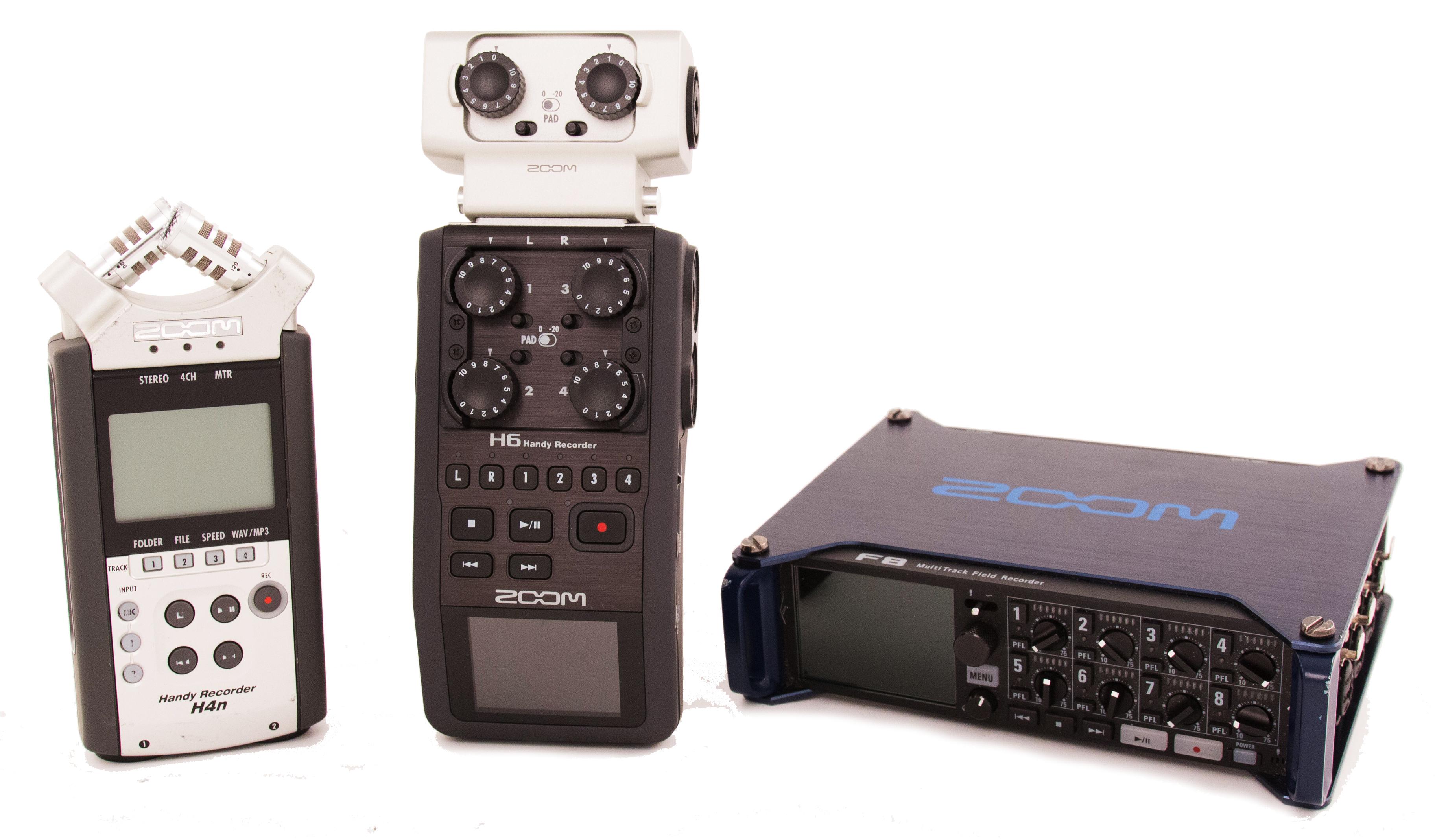The image showcases three distinct electronic recording devices, all aligned in a row. From left to right, the first device appears to be a handheld model from Zoom, vertically positioned. It has a vertical rectangular design resembling a flip phone, with a white microphone at the top, a screen, and several buttons labeled 'folder', 'file', 'speed', 'wave/mp3', and a record button, all on a silver lower half. The second device, also a handheld Zoom model, stands upright and has a black body with a white microphone head, giving it a robot-like appearance. It features various dials and controls, looking somewhat like an older flip phone or compact electronic gadget. The third device, placed horizontally to the right, is a larger desktop model, roughly the size of a VHS tape in width and about twice as tall. It boasts a screen, an array of knobs across its surface, and prominently displays the word "Zoom" in blue font on the top. The devices are primarily black and silver with the text in blue and white, likely intended for media or transmission purposes.